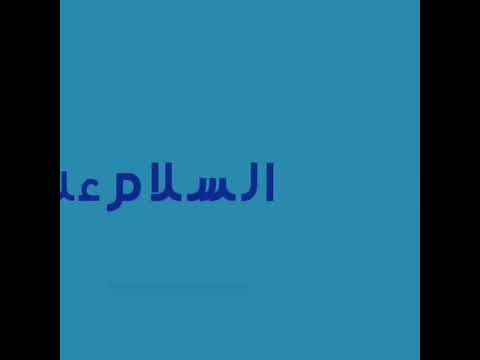The image features a blue square background with a mix of lighter aqua blue and bluish-green hues. Overlaying this background, there is a sequence of text written in a dark blue color. The text, which seems to belong to an unfamiliar or foreign language, perhaps resembling hieroglyphics or possibly even a Middle Eastern script, consists of approximately six distinctive characters. These characters include shapes reminiscent of a C, P, U, W, J, and I, and are positioned off-center to the left, with the "I" reaching towards the center of the image. On each side of the blue square, there are black vertical stripes, framing the text and adding to the visual contrast. The overall composition gives an impression similar to retro graphics from old Nintendo or Atari games.